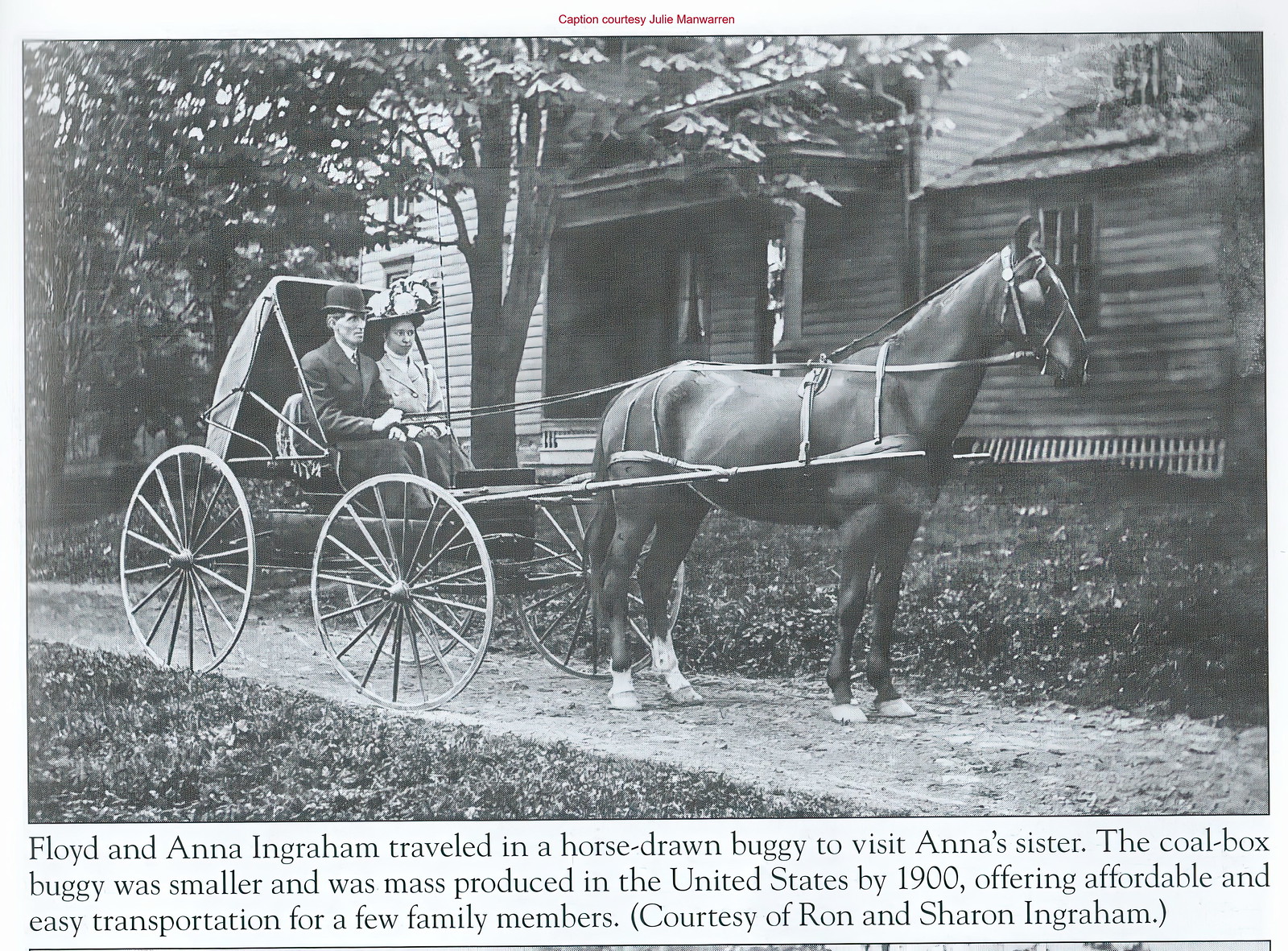In this black-and-white photograph, a horse is harnessed to a vintage coal box buggy, standing still on a dirt lane in front of a house surrounded by trees, leaves, and grass. The buggy, with its tall, thin wheels, is an example of an early 20th-century mass-produced, affordable, and smaller mode of transport. Inside the open carriage are two somber-looking individuals dressed in formal attire: Floyd Ingraham, donning a black top hat, and Anna Ingraham, wearing a highly ornate floral hat. The well-cared-for horse is adorned with numerous wires and lines on its face and an eyepatch to keep it calm. The caption at the bottom reads: "Floyd and Anna Ingraham traveled in a horse-drawn buggy to visit Anna's sister. The coal box buggy was smaller and was mass-produced in the United States by 1900, offering affordable and easy transportation for a few family members," provided courtesy of Ron and Sharon Ingraham.